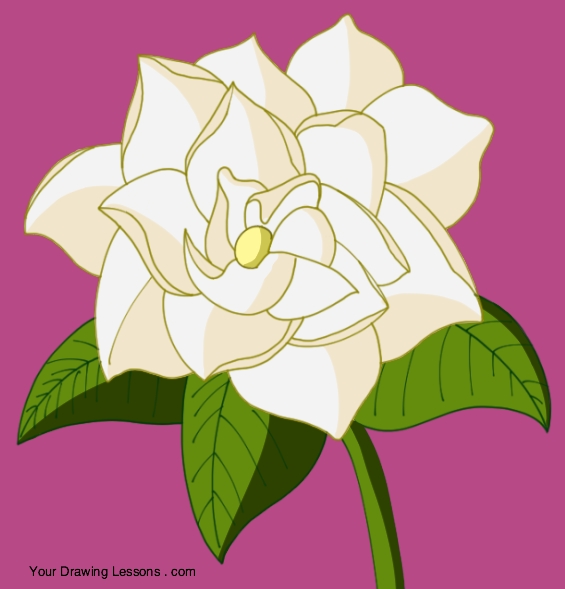The image features a digitally created, cartoon-style drawing dominating the frame, set against a solid dark pink background. Central to the image is a large flower with predominantly white petals and a yellow stamen at its center. Beneath the flower, three green leaves with visible veins spread out, while the stem extends from the bottom. The only text visible is "YourDrawingLessons.com" located in the bottom left corner. The composition and vibrant colors, including shades of green, yellow, white, pink, tan, and black, give it an illustrative feel akin to something from a coloring book.